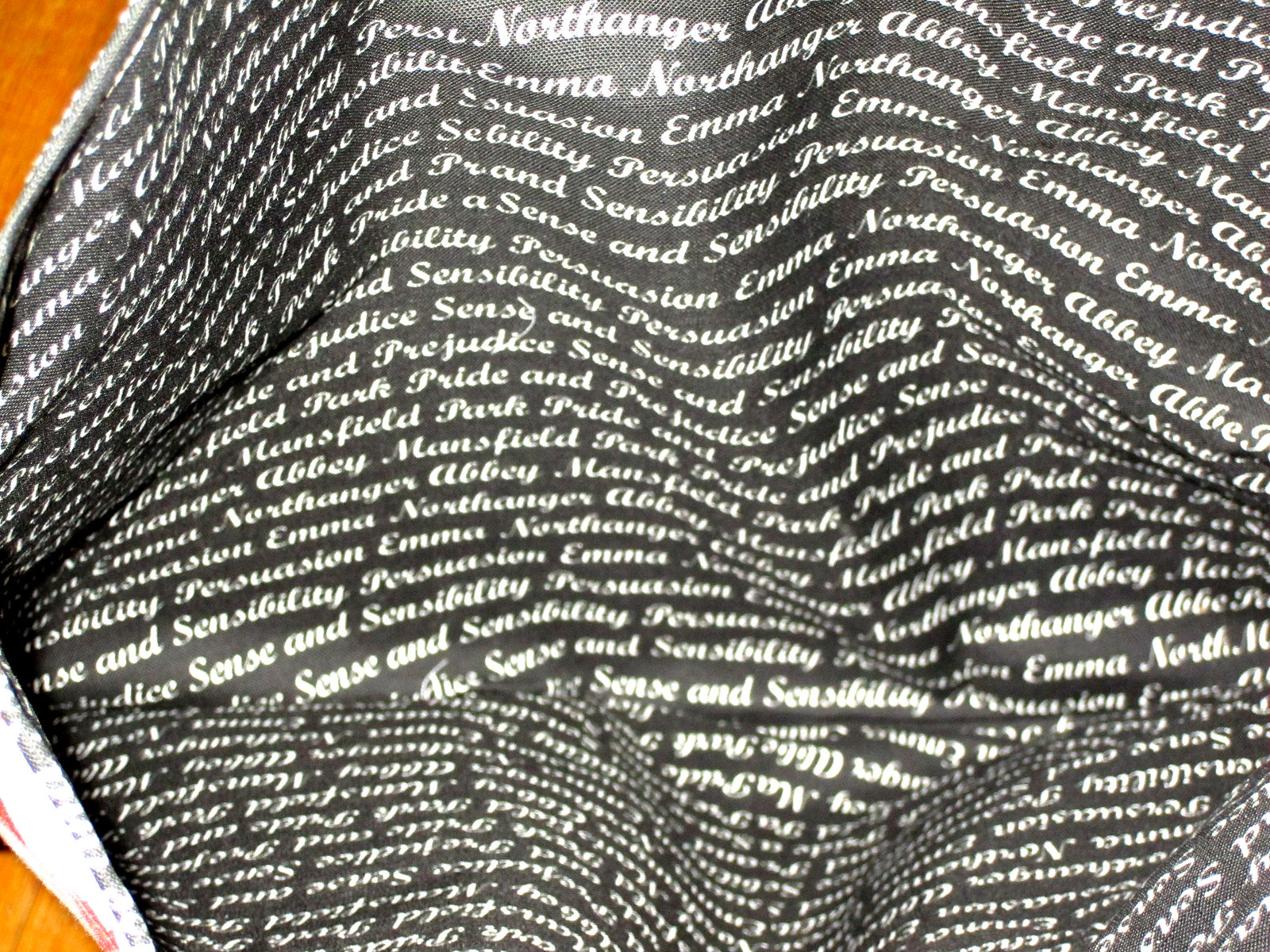The photograph features an extremely zoomed-in view of a black piece of fabric or material, possibly a bag or a piece of clothing, that is crumpled and laid out on a brown table. This fabric is adorned with small, white cursive text that is horizontally aligned and displays a repetitive pattern of words. Notable words repeated throughout the material include "Emma," "Abby," "persuasion," "manifested," "pride," "sense," "prejudice," "Emma Northinger," "Abby Mansfield," and "Sense and Sensibility." The backdrop of the fabric is black, with a sliver of golden-brown visible at the top and bottom left corners of the image.